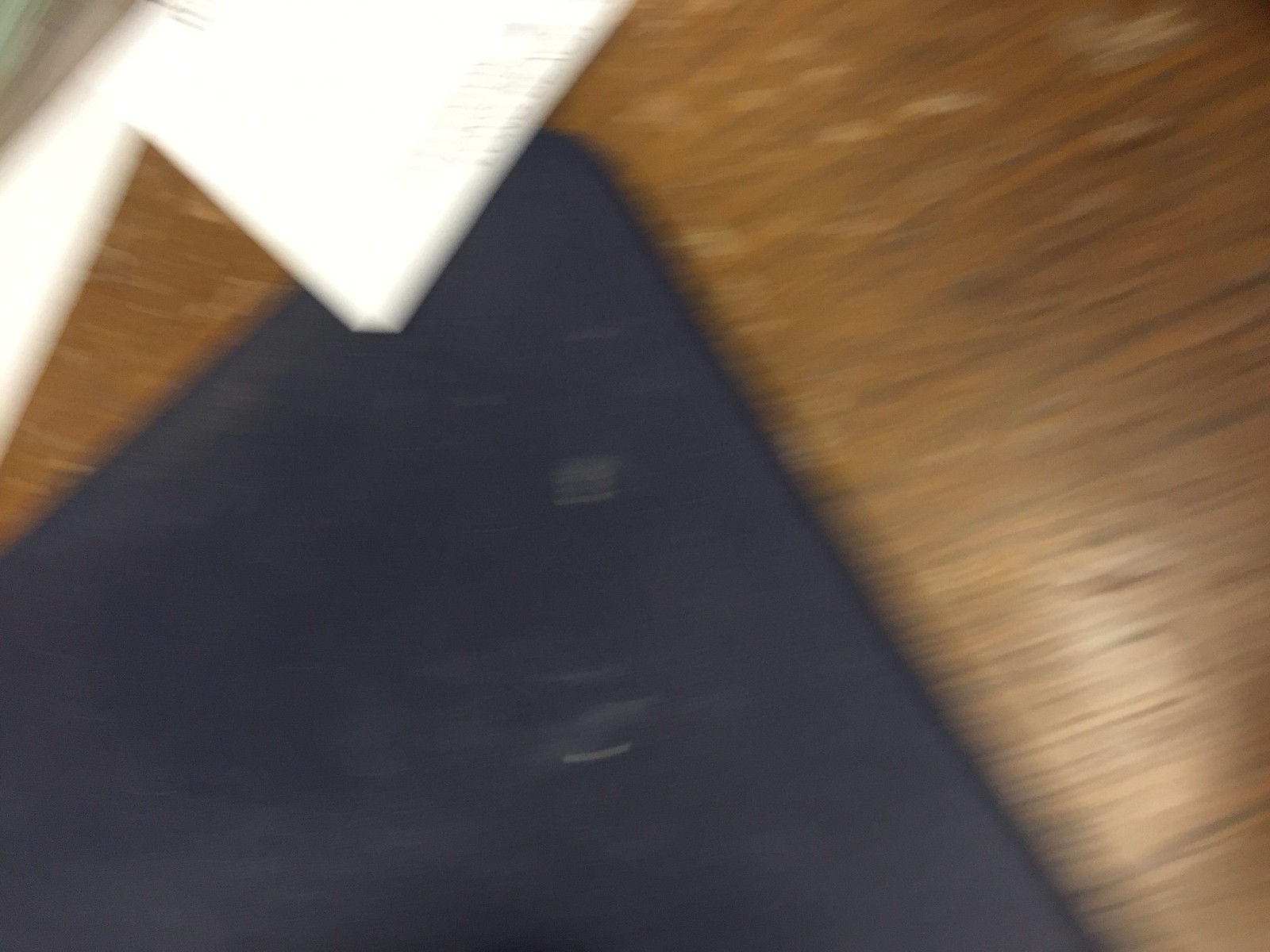This blurry photograph features a medium brown wooden surface, likely a floor or table, with black and dark brown striations running across it and visible nicks. Positioned prominently, a black triangular item extends from the center left towards the center of the image, showing lighter colored marks, possibly stains, in gray and brown hues. In the upper left corner and extending slightly downwards, an angled white surface resembling a flap or piece of paper is visible, with a shadow beneath the black triangular object. The wooden surface also exhibits scratches, especially towards the upper section. Overall, the blurriness of the image obscures finer details, but the primary elements of wood, black object, and white material are clear.